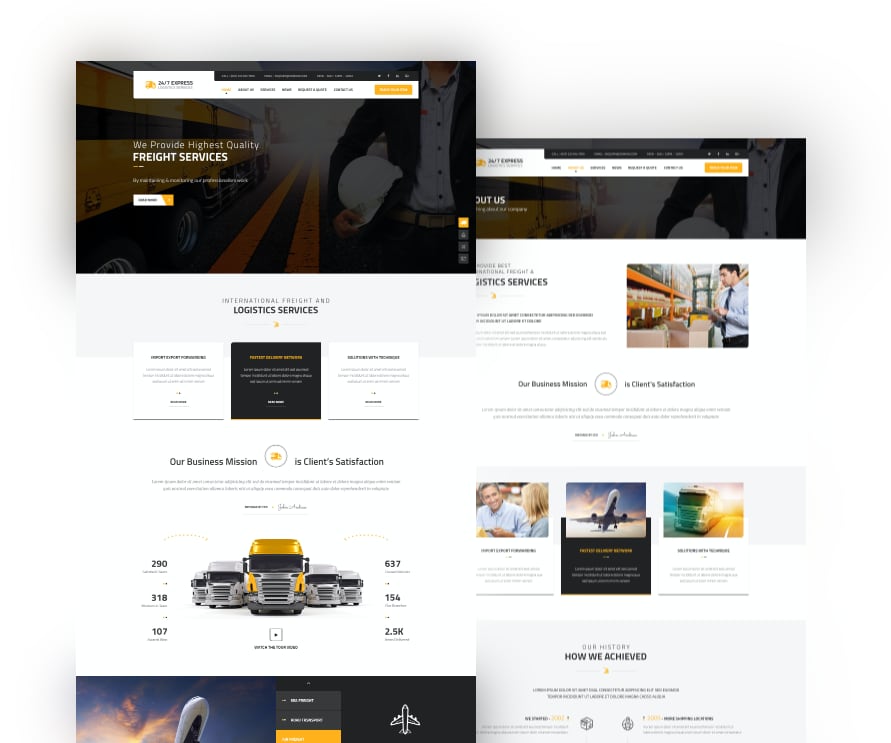The image contains two vertically stacked screenshots, likely from a logistics service company's website, and two tabs to the right that are too small to decipher. 

The top screenshot features the company's name, "24-7 Express," on the left. Surrounding the name are several tabs that are hard to read due to their small size. Below the company name is the tagline: "We provide the highest quality freight services," set against a predominantly dark background. In this section, there's an image of an eight-wheeled truck painted in yellow and black, driving on a road with dual yellow lines converging toward the horizon. There is also a partial image of a person holding a white hard hat, cropped at the head.

The lower part of the top screenshot has a white background with the text: "International freight and logistics services," followed by the company's mission statement, "Our business mission is client satisfaction." Adjacent to this text are images of a yellow truck and a cutaway view of an airplane soaring through cloudy skies.

The second screenshot, positioned to the right, appears to be the "About Us" section of the same company's website. It prominently displays the statement, "Our business mission is client satisfaction," in the middle. At the very bottom, the text reads, "Our History: How we achieved this," suggesting a narrative about the company's journey and achievements.